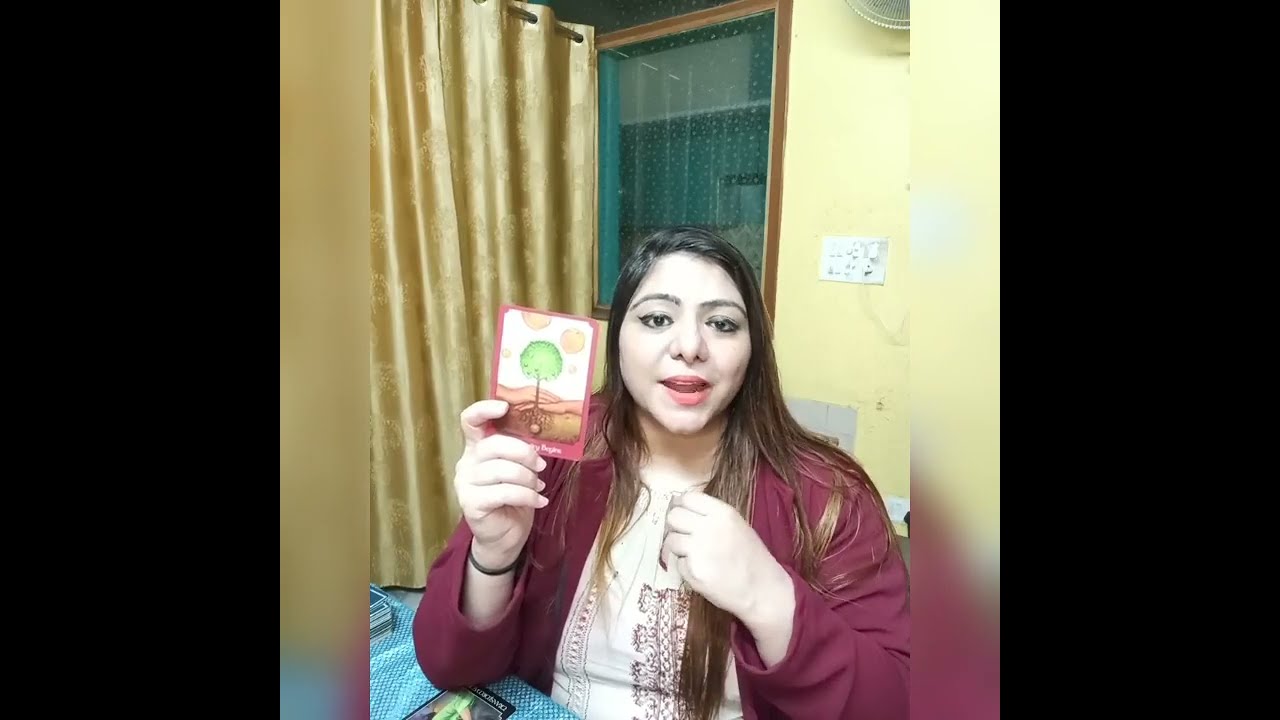The image depicts a young woman with long brown hair, darker at the roots and lighter towards the ends, suggesting dyed hair that has grown out. She is seated, dressed in a maroon sweater or cardigan over a white shirt. Her right hand holds up a card featuring a tree with visible roots and two hands behind it. This card, possibly part of a tarot card set, sits against a golden background, which might be a shower curtain behind her. Her left hand rests near her neck, partially over her hair. In front of her on the table is another card and a large stack of similar cards, indicating she might be engaging in a reading or game. The background includes light yellow painted walls, lending an aqua hue. The woman's mouth is slightly open as if she's speaking, suggesting the image may be a still from a video. The door appears to be open, adding to the casual and candid nature of the scene.